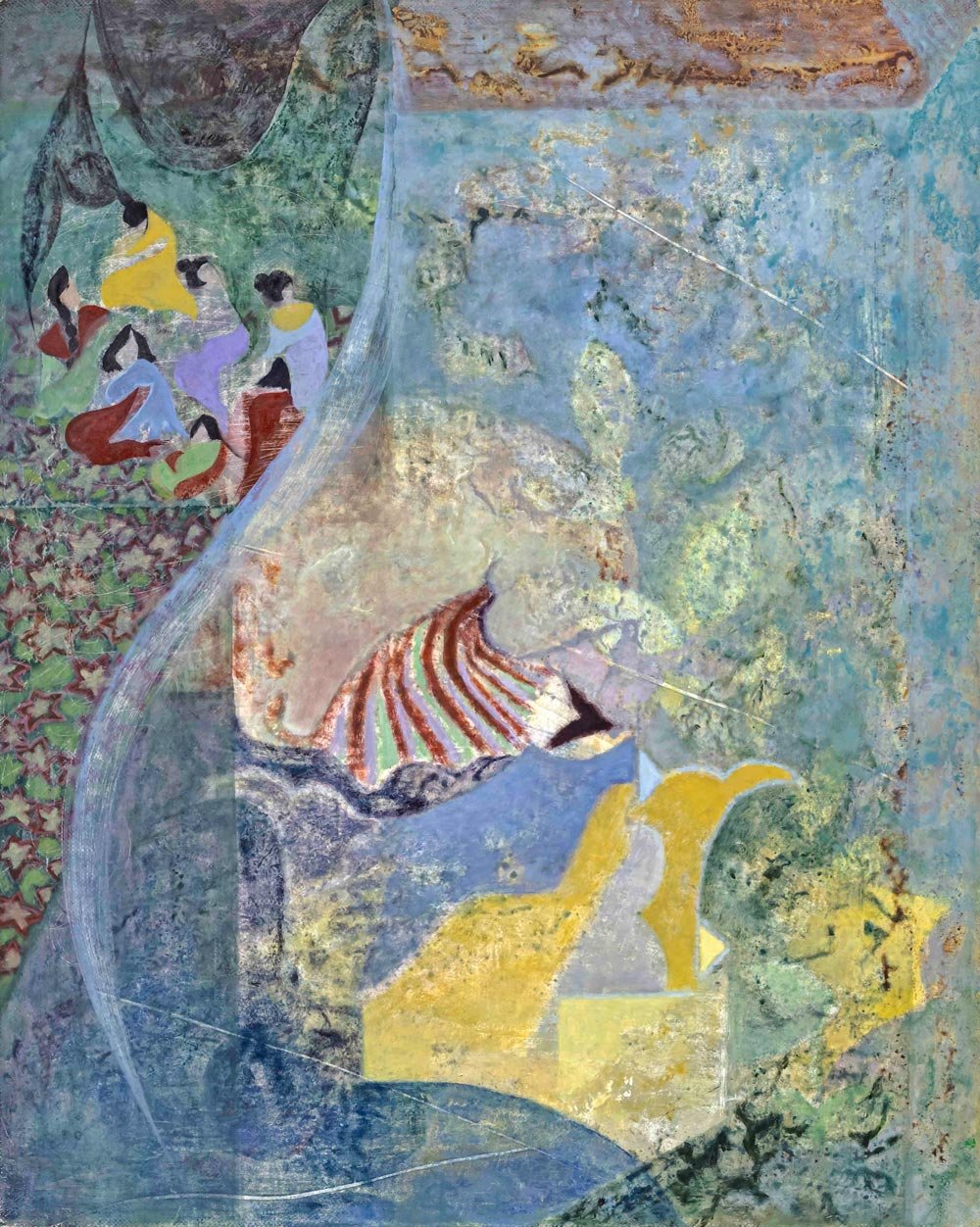The image is a textured oil painting done on a rough surface, potentially giving a bumpy feel to the touch. The top-left corner depicts a group of astonished women, their hair styled in buns reminiscent of traditional Chinese fashion. These women, possibly five in number, wear robes in varied colors including red, yellow, blue, purple, and green. Their faces are indistinct, suggesting an ethereal or faceless quality as they gaze upwards. The painting also features an extensive starry design, with numerous small stars outlined in red and filled in green, scattered below the women. Dominating a large portion of the right-hand side of the painting is a deep blue hue, descending from the top to the bottom. In the middle of the image, an individual with black hair, possibly an emperor, is seated on what resembles a golden throne, adorned in a hat. Surrounding them is a mixture of colors including a yellow shape and a red-striped tent-like figure. At the bottom, a solitary woman dressed in blue and yellow attire stands, looking outward toward the surrounding scene, adding a contemplative element to the painting. The top left corner also prominently features green and black colors, further contributing to the image’s complex and layered narrative.